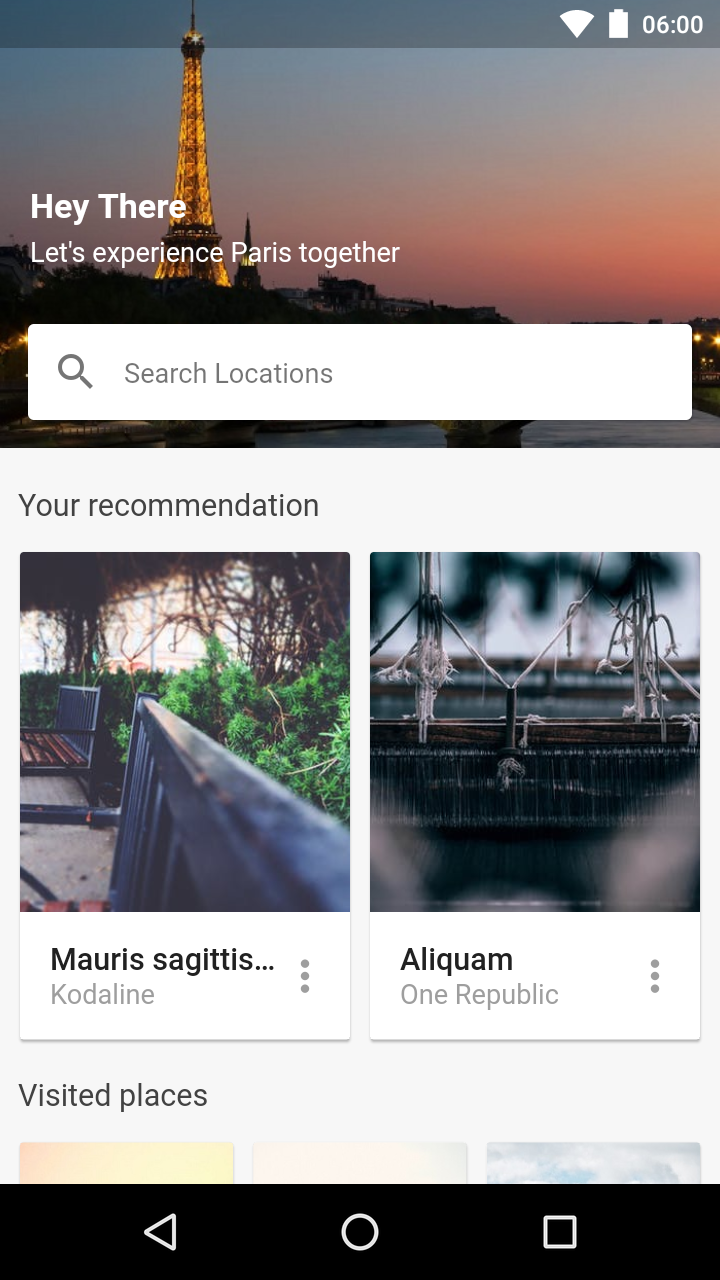The screenshot, captured on a mobile device, reveals a neatly structured application interface. At the very top, a gray status bar displays essential indicators on the right side, including the cellular signal strength, the battery life icon, and the current time, which is shown as 6:00. 

Directly beneath this bar, in the upper third of the screen, there's a captivating image of the Eiffel Tower accompanied by the enticing text, "Hey there! Let's experience Paris together." A white search bar, featuring a magnifying glass icon on its left side, lies below this image. The placeholder text within the search bar reads, "Search locations."

Further down, a section with a gray background is labeled "Your Recommendation." Within this section are two thumbnail images. The first image, situated on the left, depicts a bench surrounded by lush plants and shrubs. Below this image, the text reads "Morris Sagittus Cotoline." To the right, the second image shows ropes tied to an object, with the text "Aliquam One Republic" displayed underneath.

At the bottom of the visible portion of the screen, there's a partially cut-off section titled "Visited Places," indicating that more content lies below the current view.